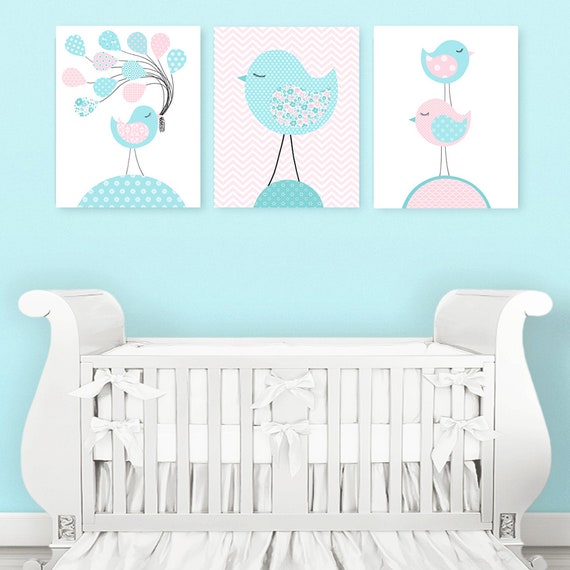This image depicts a beautifully arranged baby’s nursery with a serene light blue wall and a white baseboard. A meticulously made white crib dominates the space, featuring white sheets and white bows adorning its slats. Above the crib, three distinct paintings of stylized birds add an artistic touch to the room. 

The left painting showcases a light blue bird, matching the wall color, facing right and holding several colorful balloons, with a pink wing. The center artwork mirrors the wall color with a bird facing left, its wings embellished with light blue and pink dots, standing on a half-circle. The rightmost image presents a whimsical depiction of two birds stacked atop one another. The upper bird, light blue with pink wings dotted in white, faces right, perched on a pink bird with light blue, white-dotted wings that faces left. 

The harmonious blend of the light blue and white theme, complemented by the delightful bird illustrations, creates a tranquil and charming atmosphere perfect for a baby’s room.